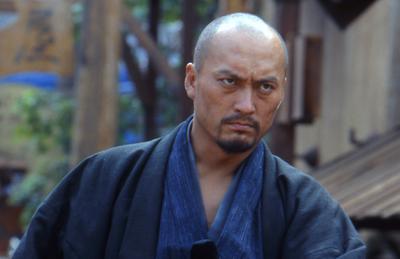The image depicts an Asian man with an intimidating and warrior-like appearance, set against a traditional outdoor scene. He has brownish skin and a bald head with a horseshoe-shaped fringe of very short, shaved hair. A goatee accentuates his fierce expression. His attire consists of a navy blue kimono with layers that include lighter blue hues. The background is a rustic, old village with prominent wooden structures: a hut on the right, a wooden building, poles with curved sections, and a sign with black Asian writing. Trees frame the scene to the left, indicating an outdoor setting during the daytime. The man, standing or possibly sitting as the image is taken from his chest up, looks off to the right, away from the camera. Various colors are evident in the image, including royal blue, dark blue, light blue, green, light green, tan, white, and black, enriching the traditional and serene atmosphere.